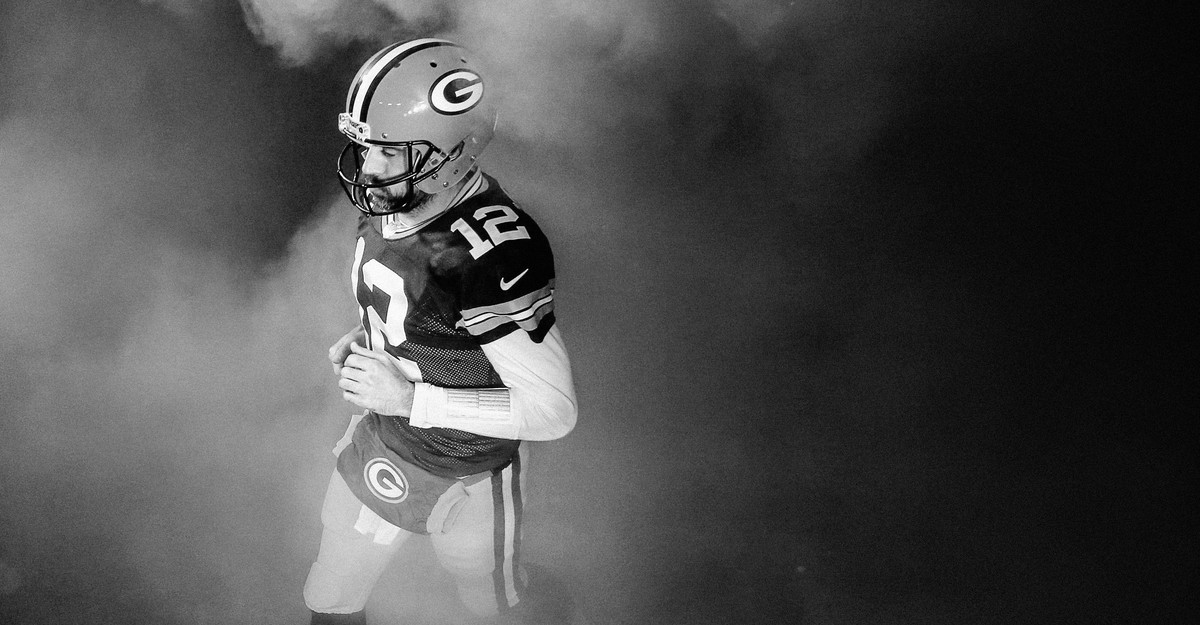This is a black-and-white horizontal rectangular photograph depicting NFL quarterback Aaron Rodgers, number 12, of the Green Bay Packers. The setting features Rodgers walking through a foggy or smoky environment, possibly enhanced by a fog machine for promotional purposes. The background is predominantly black, with a smoky white area accentuating the left side. Rodgers appears expressionless, donning his complete game uniform, which includes the Packers' iconic jersey, helmet emblazoned with a large "G" logo, and pants. He has a beard and mustache, wears a white long-sleeve shirt under the jersey, and sports a hand muff around his waist with another "G" logo. The Nike logo on his jersey is also visible. His hands are positioned in front of him, not holding a football, and the image captures him from head to knees. The photograph's dramatic use of light and shadow, combined with the element of mist, lends an evocative and almost ethereal quality to the shot.